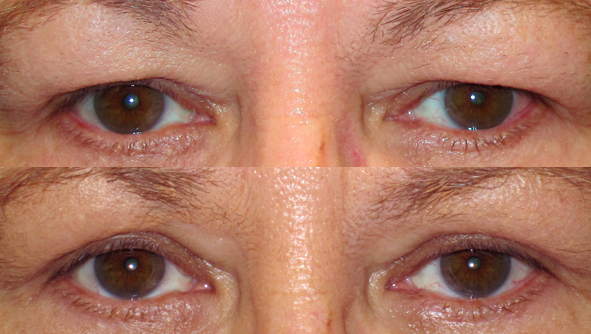This is a close-up, horizontally bisected image focusing on the eye region of a person with brown eyes and brown eyebrows. The photo showcases a "before and after" scenario with two sets of identical features, one above the other. Both sets contain the bridge of the nose, the eyes, and the eyebrows within a narrow strip. The top image displays eyelids with a pinkish hue, while the bottom image reveals more clearly defined eyelids with a more pronounced pinkish or bruised look around the eyes. A notable mark is present on the right side of the bridge of the nose in both images, reaffirming that they belong to the same person. The consistent details and the subtle changes between the two layers highlight the intended purpose, likely demonstrating a cosmetic or medical alteration.